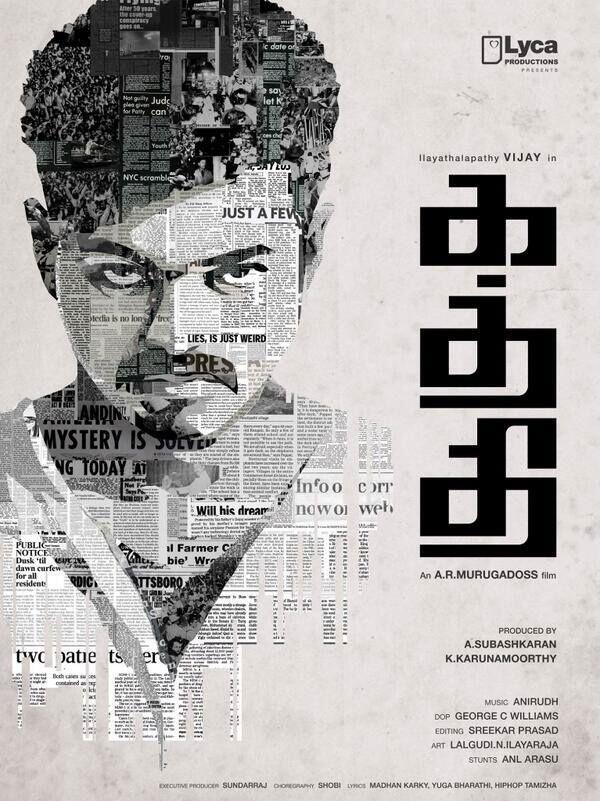This image is a highly detailed, black-and-white poster, potentially an advertisement for a movie, with text written in an Indian or Near Eastern language. The central feature of the poster is a striking collage of a young man, whose face, neck, and torso are meticulously crafted from English newspaper clippings. These clippings include phrases like "lies is just weird" and "mystery is solved," among other fragmented texts. The man has prominent facial features including intense eyes and a mustache, and his direct gaze appears to engage the viewer. At the top right corner of the poster, it says "Laika Productions" followed by a foreign name in a large font, possibly in the same Indian or Pakistani script. The names "A. Subhash Karan" and "K. Karuna Murthy" are listed at the bottom, credited as producers. The overall aesthetic underscores the creative effort behind the artwork, blending traditional portraiture with modern collage techniques.